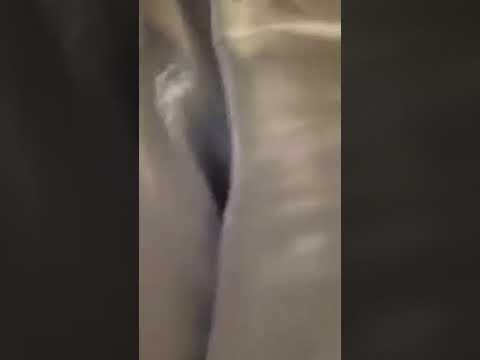The image is a very close-up, blurry view of what appears to be two columns or folds of a taupe or light brown fabric, reminiscent of silk, with a dark, vertical gap or line separating them. The columns are light-skinned toned and touch at the bottom, overlapping slightly, while they are more spaced apart at the top, revealing a dark grey to black area in between. There is some shimmering or white highlighting on the surface of the columns, adding to the difficulty in making out clear details. The background at the bottom of the image is dark grey, and the entire scene is framed by a vertical rectangle. The image might be a painting or an abstract representation, and its blurred, super-zoomed quality leaves much to the viewer's interpretation.